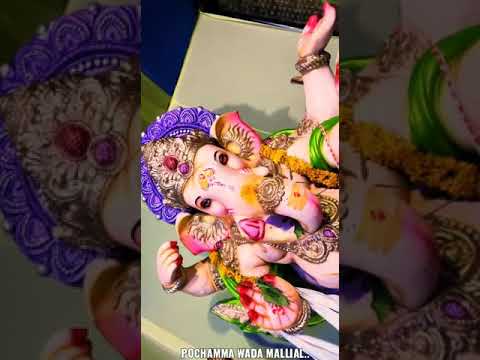The image depicts a detailed and ornate statue of an elephant-like figure, seemingly inspired by Hindu iconography. The central focus is on the lighter area of the figure, which features the head of an elephant adorned with intricate decorations. The head is positioned in the middle-left of the image, angled sideways with the trunk pointing to the left and the body extending to the right. The skin of the elephant is a pale pink color, with a brighter pink hue on the trunk.

The figure wears a lavish headdress composed of a golden crown adorned with red and purple jewels, atop which is a purple crown that radiates as a wreath resembling petals or flowers. The crown and wreath add to the statue's rich visual complexity. The figure also features an unusual blend of human-like elements; it has multiple arms—specifically, three visible arms each with human hands adorned with red nail polish. One hand is extended outward with its palm facing up, another is curled forward, and the third, in the foreground, mimics a stop sign gesture with a leaf detail on the palm.

The elephant’s body is embellished with various forms of jewelry, including gold pins and necklaces. It has painted floral motifs, such as a yellow flower on its trunk and suns emanating from its ear. At the bottom of the image, there is an inscription in an unfamiliar script, which reads "Pokamawaramaleel." The background features shaded rectangular areas on the right and left, framing the central, well-lit figure.